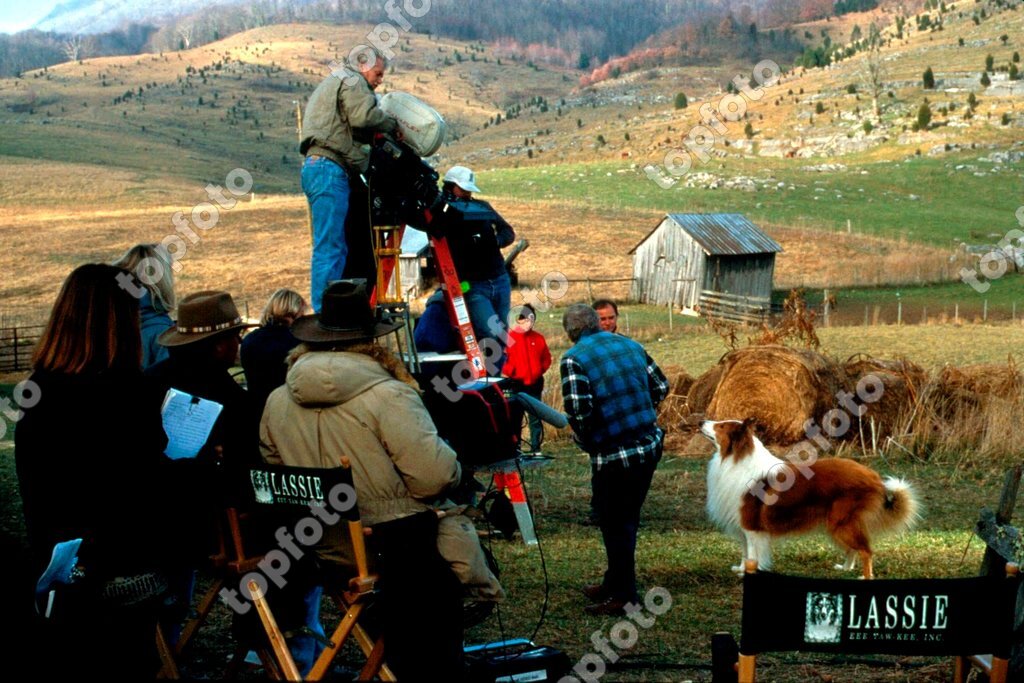The image is a behind-the-scenes photograph of a movie set, presumably for a film featuring the famous collie, Lassie. The scene is set outdoors with a picturesque background of rolling hills covered with green grass, high mountain ranges, rock cliffs, and a mix of tan and green fields, suggestive of farmland or cropland and further accentuated by a fenced farmland with a barn and shed. The photograph, in a horizontal rectangular format, is watermarked diagonally with semi-transparent text reading "Top Photo." 

In the foreground, people are bundled up in parkas, flannel shirts, and some are seated in foldable director's chairs that have black fabric seats and backs. A prominent chair in the bottom right corner has the name "Lassie" printed on it. Standing nearby is a man dressed in a blue plaid vest over a black plaid long-sleeve shirt and black pants, looking down at a dog that closely resembles Lassie, with a brown body, white mane, and a white spot on its face.

A camera is mounted on top of a ladder, pointed out over the expansive field, capturing the scenic backdrop and the activities on set. The presence of multiple people observing the scene, sitting in similar chairs, reinforces the bustling atmosphere typical of a movie set. The scenic beauty, detailed landscape features, and the watermark contribute to the authenticity of this behind-the-scenes glimpse into the timeless classic, Lassie.